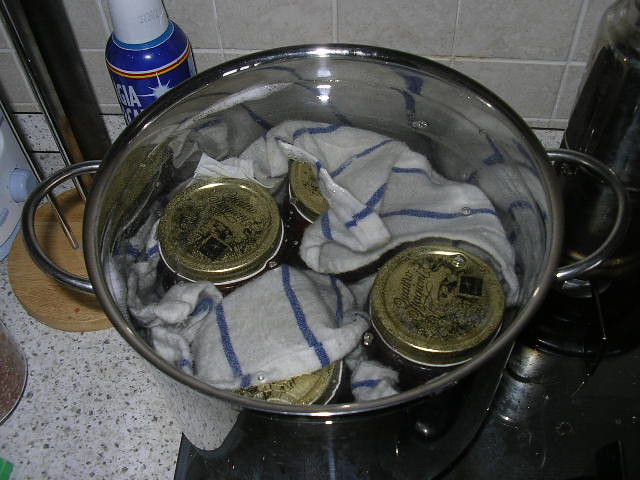This image is a low-quality, flash-taken snapshot of a kitchen counter and stove, viewed from above. The counter is speckled granite in shades of white, brown, and gray, and it sits against a beige tiled wall. Dominating the scene is a large, tall stainless steel stock pot with two silver handles. Inside the pot, several mason jars with gold lids featuring black text and illustrations are partially submerged in water. The jars are surrounded by white and blue striped dish towels. To the left of the pot, there is a blue spray can with a white cap and a label displaying the letters "GIA" in white text along with some other obscured letters. Nearby, a dish rack holder sits empty. Additionally, part of a toaster is visible near the left-center of the image. The image captures a domestic setting with an assortment of kitchenware and household items scattered around.